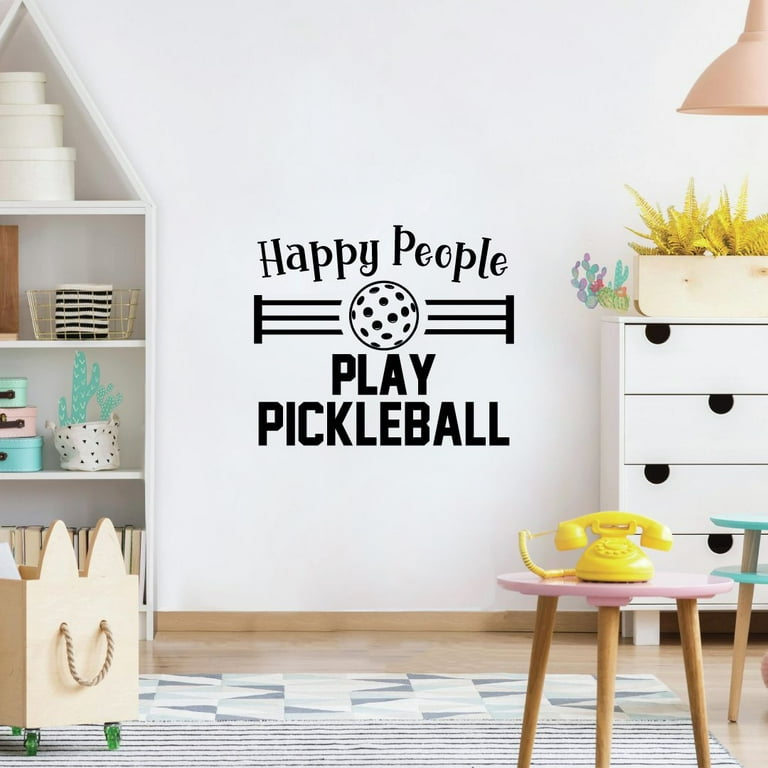This detailed color photograph captures a cheerful and well-organized child's playroom. The back wall is crisp white and features a black stencil that reads "Happy People Play Pickleball." The words 'Happy People' are in a playful black font with capital H and P, and below, 'Play Pickleball' is bolded in all caps. Centered between the text is an animated black pickleball net holding a white ball with black holes.

On the left side of the room, a bookshelf with a triangular peak has three shelves populated with various items. The top shelf holds three small circular hat boxes in increasing size from top to bottom. The middle shelf displays assorted knickknacks, while the bottom shelf houses books with their spines facing inward. A shopping bag with green wheels and a large rope handle rests on the floor beside the shelf.

On the right side of the room stands a white dresser with four staggered drawers, featuring cut-out handholds for easy opening. Atop the dresser sits a natural wooden plant container with vibrant yellow spiky leaves. Partially visible above the dresser is a pink hanging lamp. 

In the foreground, a small three-legged table with a pink top holds a vintage yellow rotary phone. There’s also mention of another table with a turquoise top partly cut off by the edge of the photo. The floor is hardwood with a stylish gray and white rug featuring blue triangles and stripes. Additional details like the natural brown wall molding and muted but cheerful color scheme add to the room's inviting ambiance.